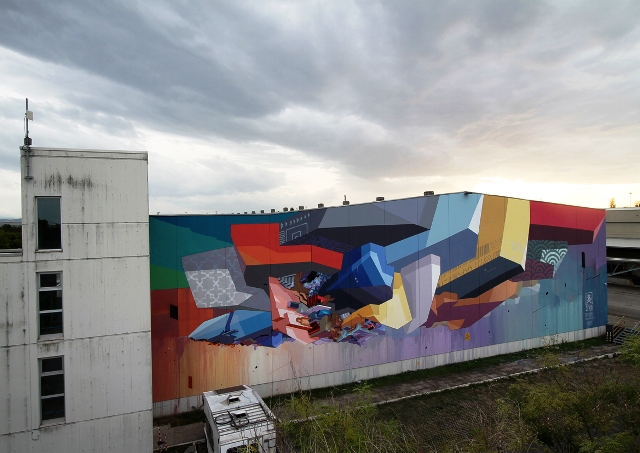This image captures a vivid, abstract mural painted on the side of an old, possibly abandoned factory building situated in a somewhat industrial area. The mural, which showcases an array of bright and bold colors including red, blue, yellow, and orange, features a mix of shapes like rectangles and squares. The artwork transitions through a spectrum of colors, starting with green on the top left and blending into blue, red, gray, lighter blue, and yellow. Below this colorful medley, the design evolves into a brilliant rainbow gradient moving from red and orange through brownish tones to purple and various shades of blue. In front of the mural, overgrown grass adds to the sense of neglect, while cloudy, gray skies form a moody backdrop that covers about half of the image. To the left of the mural stands a three-story structure characterized by a simplistic white facade and three windows per floor, possibly indicating an old staircase area.